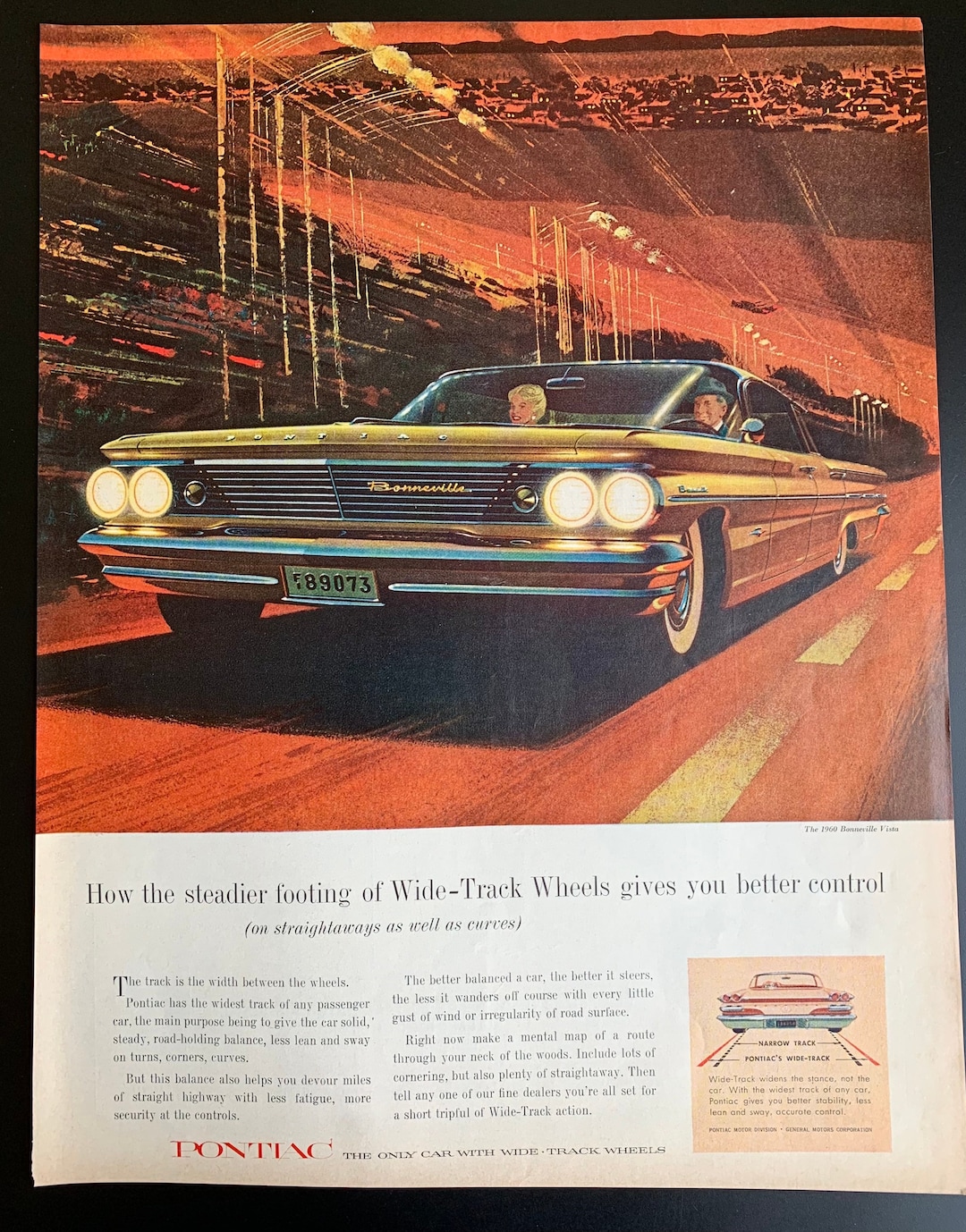The image is an illustrated advertisement poster from an old magazine featuring a Pontiac Bonneville. The car, depicted in a golden-yellowish hue, is prominently shown from the front and side, appearing to race down a highway with an emphasis on speed and control. It has four doors and notable fin-like extensions on the back. The front of the car showcases two circular headlights on each side and a smaller third headlight near the grill, which is crafted from stainless steel, complemented by a stainless steel bumper and white wall tires.

In the car, a man wearing a hat is driving, while a woman with blonde hair and large earrings sits beside him. The background consists of rich reds, browns, and oranges, suggesting a dynamic, possibly hilly landscape with a town visible beyond. The car and its passengers are depicted in a stylized, cartoon manner.

At the bottom of the poster, there's text explaining the benefits of the car's wide track wheels in providing better control, accompanied by a diagram illustrating the positioning of the wheels on the road. The advertisement prominently features the Pontiac name along the bottom.